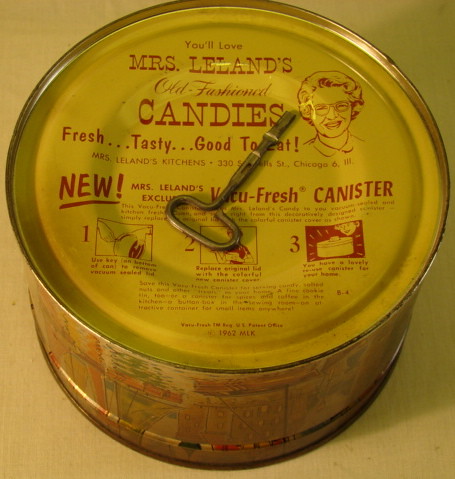This image showcases a vintage can of old-fashioned candies, likely from the 1970s or 1980s. The can is predominantly yellow with red lettering, sitting on a beige countertop. On the top of the can, there is a metal pull tab designed for opening, and instructions about how to use it. The text reads, "You'll love Mrs. Leland's old-fashioned candies. Fresh, tasty, good to eat." It includes the details of "Mrs. Leland's Kitchens" along with an address in Chicago, Illinois. Adjacent to the text, there's a picture of Mrs. Leland, an elderly lady with glasses and white hair, who appears to be in her 80s or 90s. The can has a decorative edge that features watercolored houses and trees. Despite its old appearance, the can seems to be a new item and boasts a "vacuum fresh canister" marked as a Mrs. Leland's exclusive.